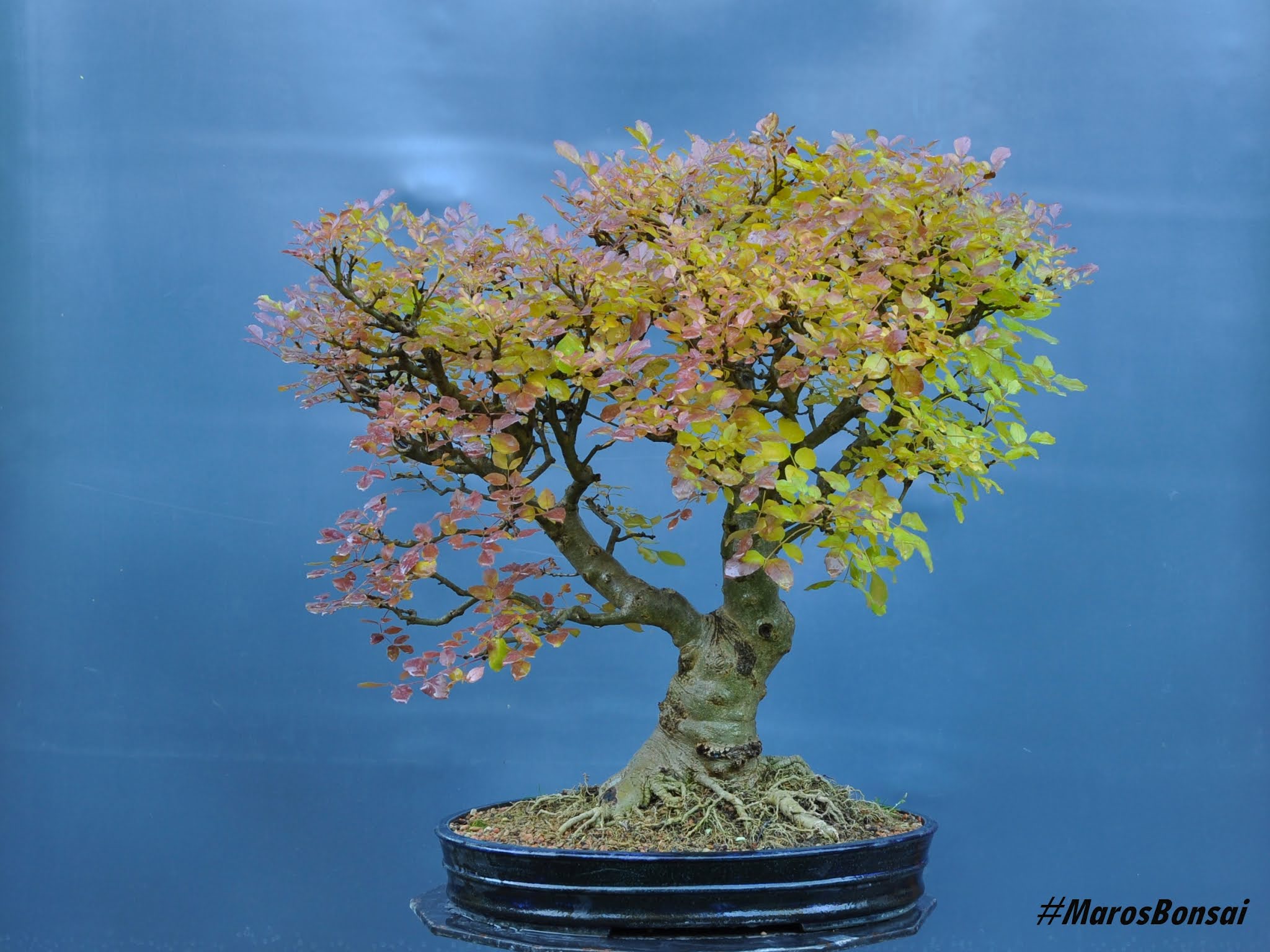In this picture, you see a beautifully groomed bonsai tree with a thick trunk, sprouting several branches adorned with vibrant foliage. The leaves are a mix of colorful hues—light green, pink, and a touch of orange. The tree is planted in a shallow, circular-shaped blue flower pot, with some of the roots visibly emerging from the soil. The background of the image is an airy blue, further enhancing the vividness of the bonsai. In the bottom right corner, there is a watermark that reads "#MarosBonsai" in black letters.